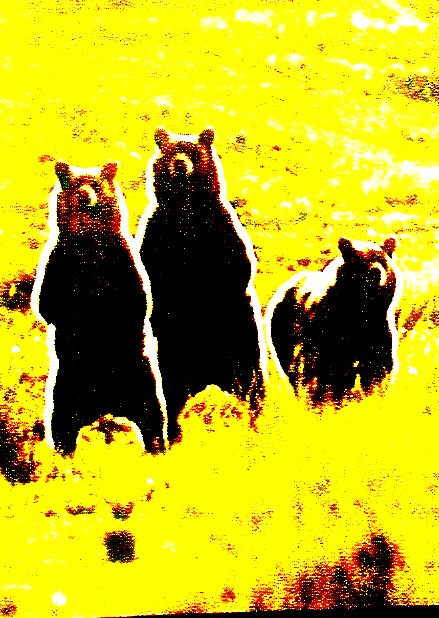This image appears to be a digitally altered photograph featuring three brown bears in a field with a vivid, almost fluorescent yellow background. The composition shows two bears standing upright on their hind legs, with the taller one positioned to the right of the slightly shorter bear. To their right and slightly behind, a third bear is on all fours, seemingly in motion and looking in a different direction than the other two. The bears are dark brown with lighter brown heads, black noses ringed with yellow, and ears sticking straight up. A noticeable white outline, akin to an aura, surrounds the bears, further accentuating their presence against the distorted, grainy backdrop. The background, which includes a hillside, is predominantly yellow with white splotches and hints of brown and tan. Overall, the image possesses an infrared-like quality that enhances its surreal and striking appearance.